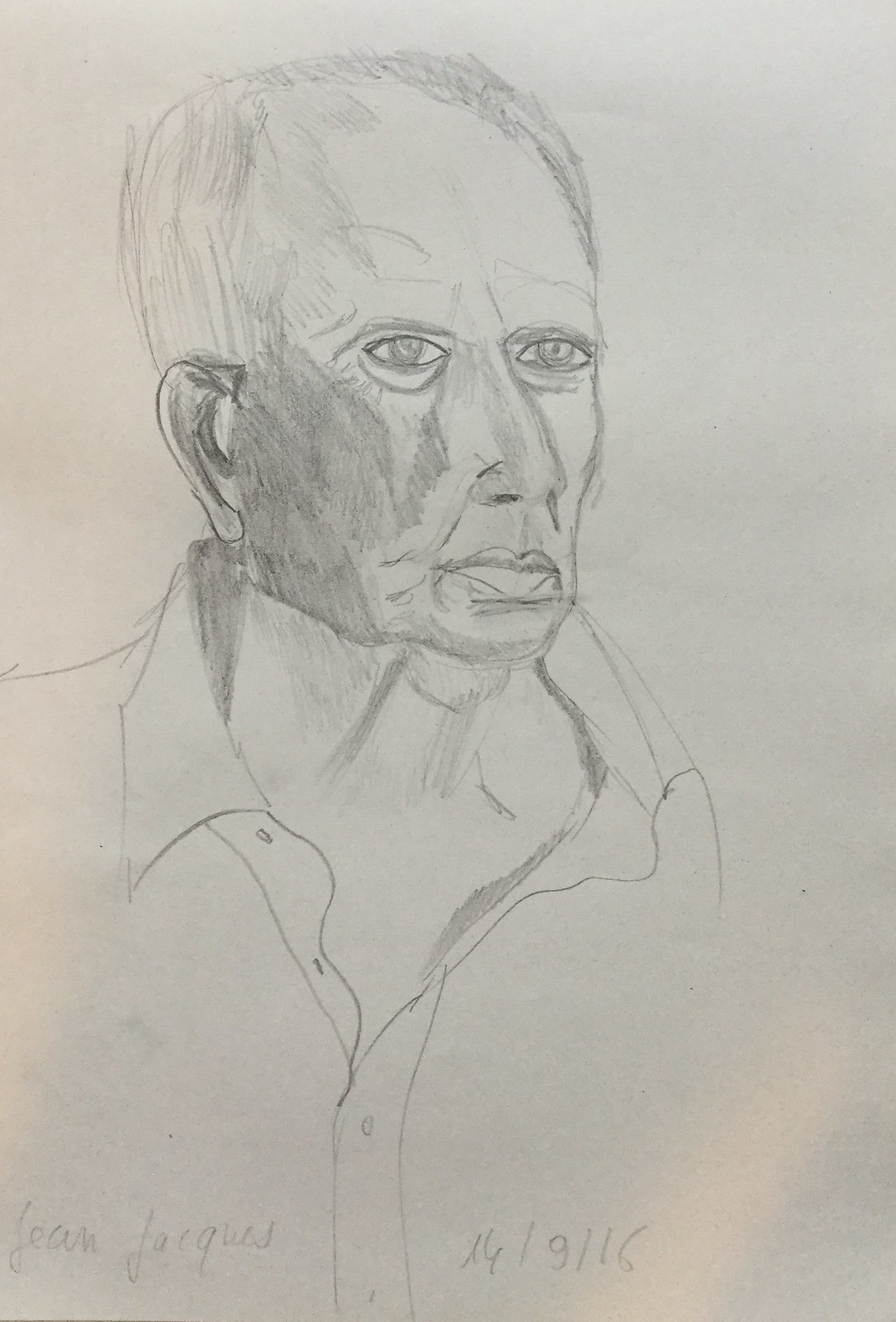This detailed pencil sketch, created on a pristine white sheet of paper, features a close-up portrait of an elderly man. The drawing is so large that it dominates the entire visible area, with no paper edges in sight. The man, who is balding on top, has sparse hair on both sides of his head. His figure is turned towards the right, offering a comprehensive view of the left side of his face, his frontal profile, and part of his chest. 

The subject is dressed in a button-up shirt, intricately rendered in pencil strokes. Expertly applied shading accentuates the facial contours, particularly along the left side of his face and ear. The artist has meticulously shaded his right nostril, giving the impression of a small drop of blood emerging. The man's weariness is palpable through the carefully drawn bags under his eyes.

At the bottom left corner, the artist's signature is inscribed in pencil, while a date is marked towards the lower right corner, anchoring the piece in both identity and time.